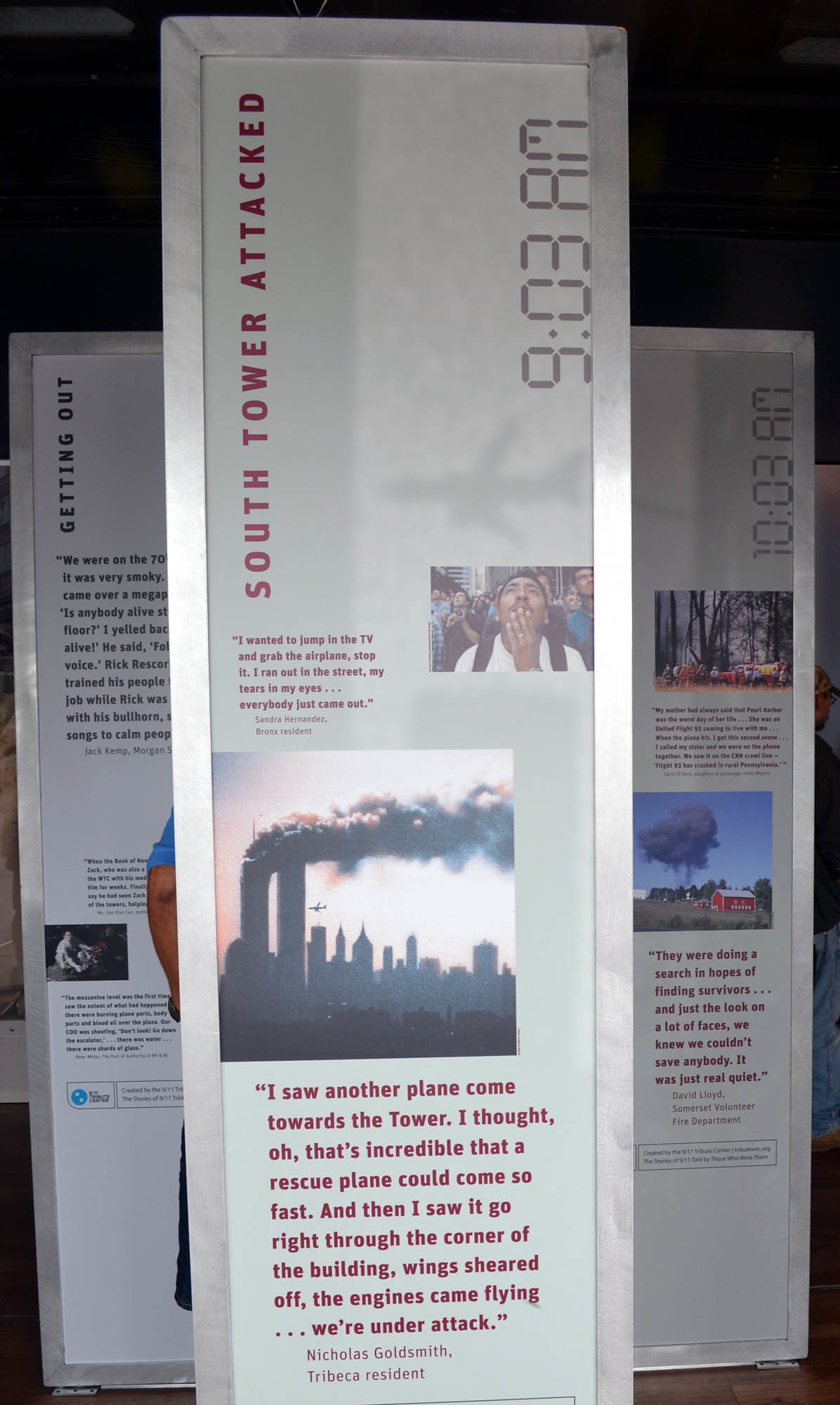This photograph, horizontally oriented and taken inside a museum, captures a tall, vertical sign commemorating the 9-11 attacks on New York City's Twin Towers. The sign reads "South Tower Attacked, 9:03 a.m." and features a series of smaller photographs and texts below it. One poignant image shows the Twin Towers engulfed in thick smoke with the New York City skyline in the background, and a plane about to collide with the South Tower. The sign includes a quote from Nicholas Goldsmith, a Tribeca resident: "I saw another plane come towards the tower. I thought, oh that's incredible that a rescue plane could come so fast. And then I saw it go right through the corner of the building. Wings sheared off. The engines came flying. We're under attack." Additional signs flank the main placard, and a person's arm is visible just behind the central exhibit, adding a human touch to this powerful tribute.